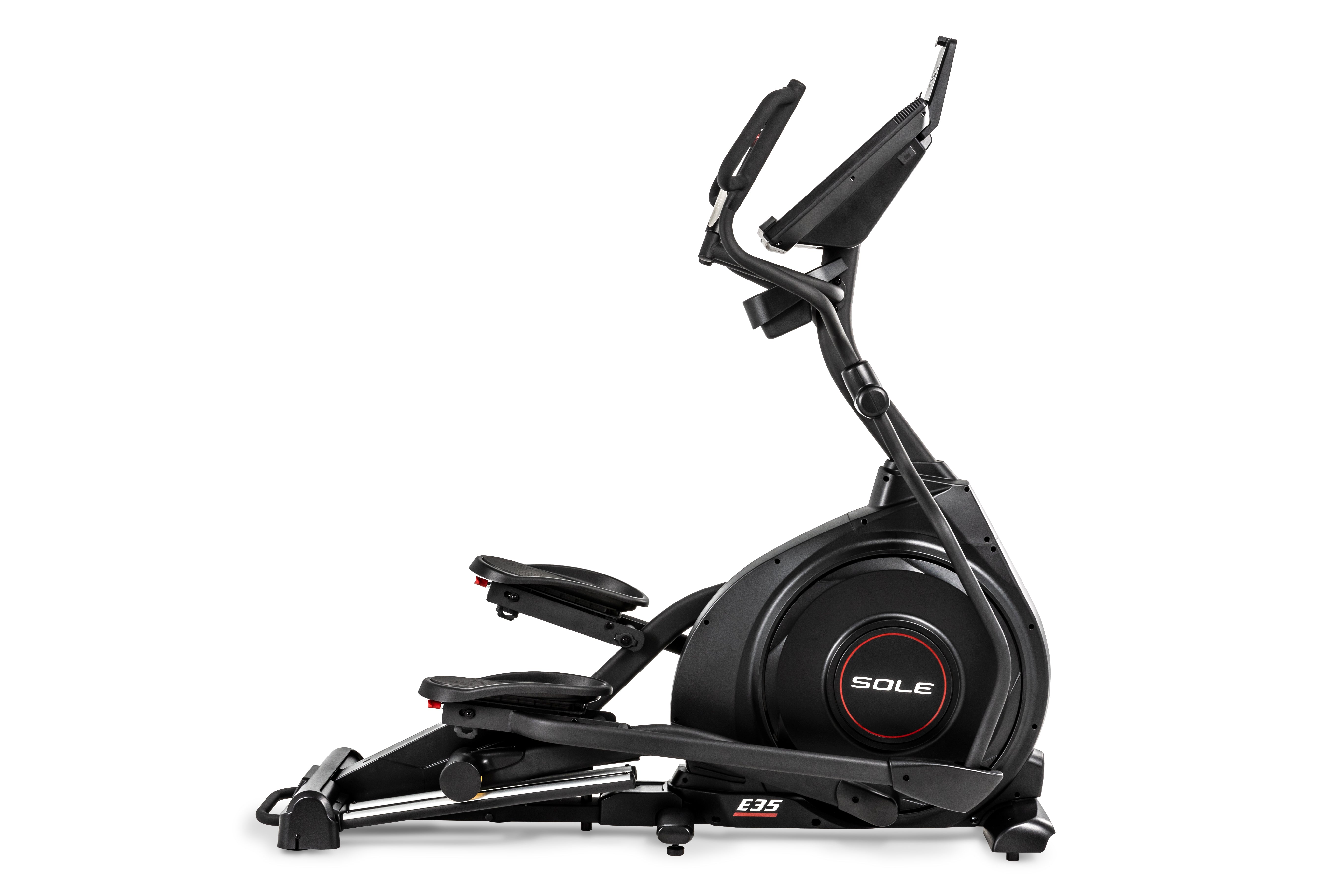The image depicts a sleek, black stair climber exercise machine set against a stark white background, likely edited for a clean presentation. The machine is predominantly black with a glossy finish and features a large screen and angled handles at the top for viewing exercise options and tracking progress. These handles, extending outward, are designed for stability and user comfort. Below the handles, the machine transitions into a sturdy circular mechanism, cobalt gray in color, with prominently displayed "S-O-L-E" in white letters, encircled by a thin red ring. Towards the base, the equipment has two designated stepping platforms for foot placement, connected to metallic, cylindrical rods for added durability. Below these platforms, the model designation "E-35," underlined in red, is visible. With its expansive base and robust side supports, this sizable piece of exercise equipment offers stability for intense workouts.